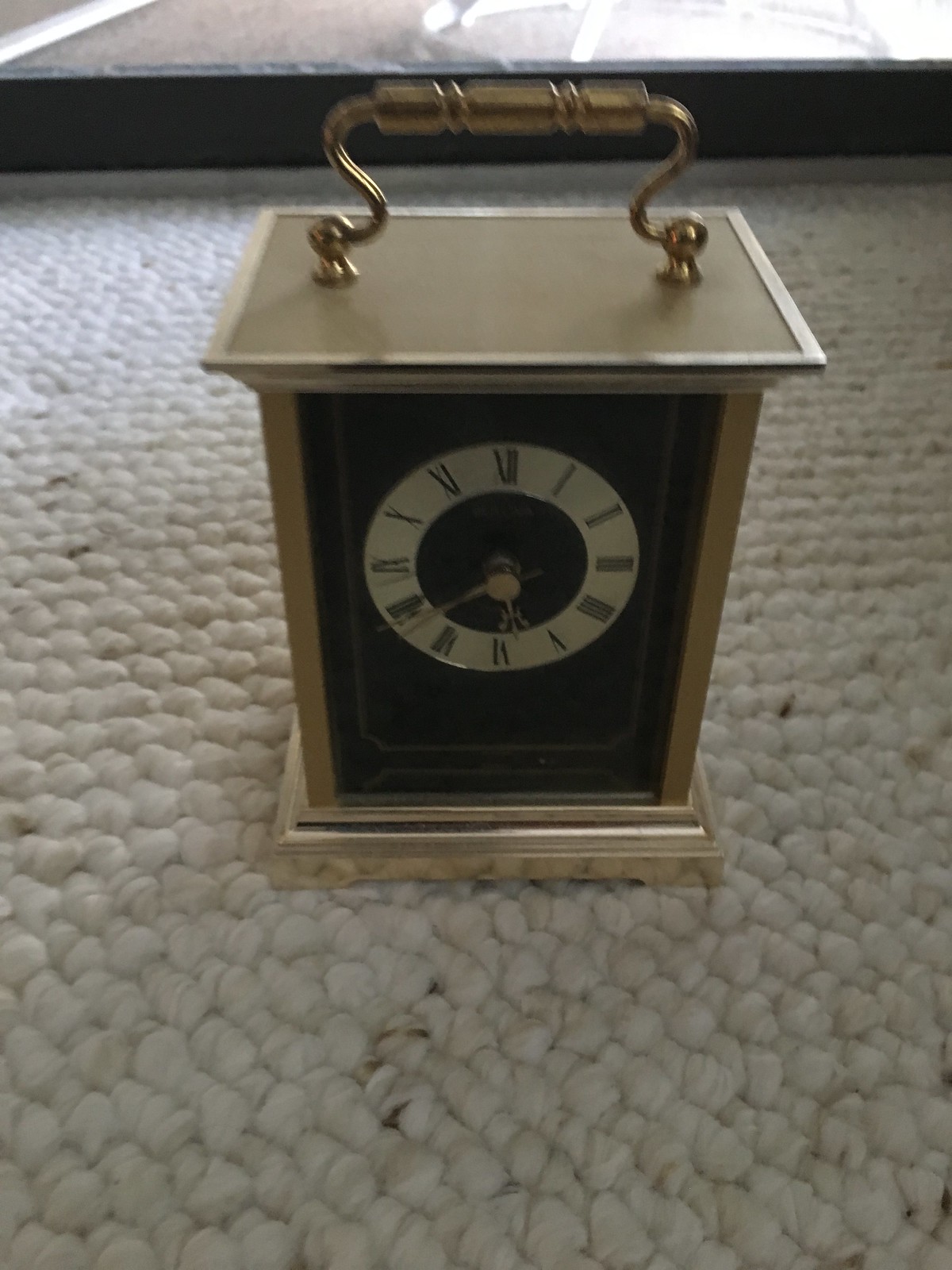In this photograph, we see a small handheld clock designed in the shape of a square lantern with a distinctive brass handle on the top that curves inward and then outward. The clock's housing is primarily a dull gold or brass-colored metal, reflecting a mix of chrome and gold hues. The clock features a rectangular face with a white circular dial displaying black Roman numerals from I to XII. At the center of this white circle, there is a smaller black circle where the golden or brass-colored hour and minute hands are attached. The base of the clock also shares this golden trim, creating a cohesive aesthetic throughout its design. The clock is placed on a large, white, shaggy carpet that appears somewhat dirty and stained, resembling popcorn or cotton in texture. Positioned behind the clock is a small podium or stand, only a few inches tall, further accentuating the clock as the main focus in the center of the image.